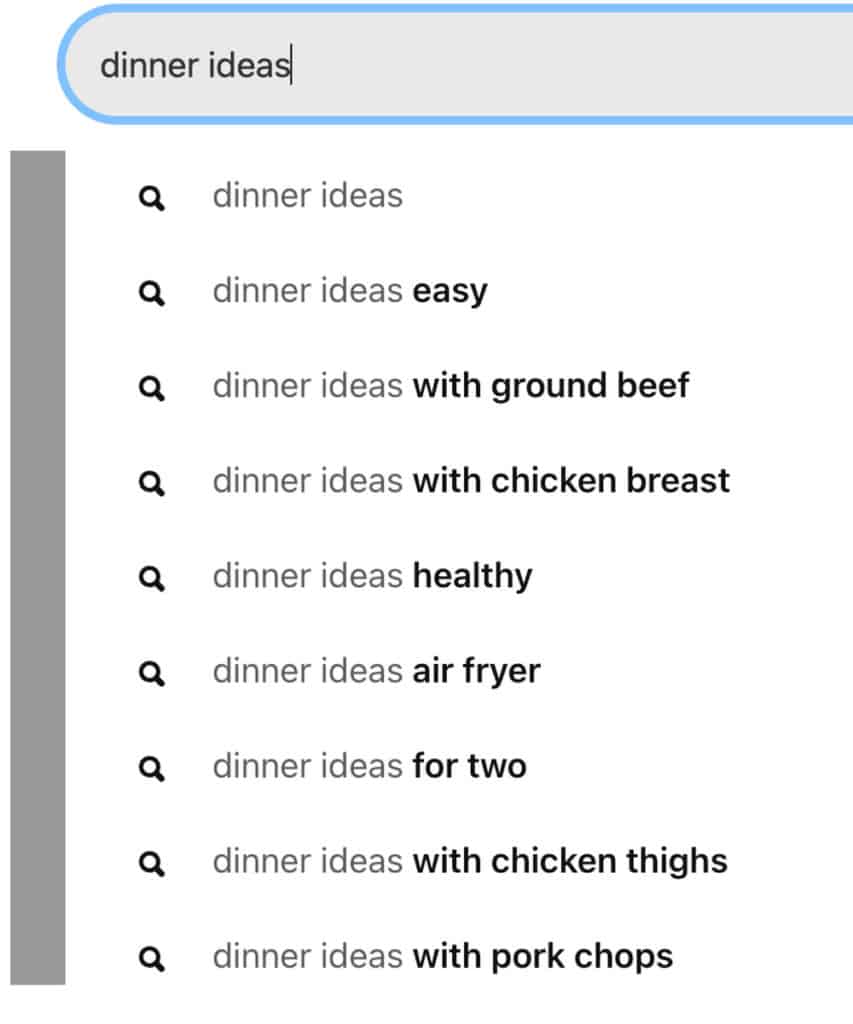This image captures a computer screen displaying a search engine results page. The search query "dinner ideas" is typed into a rectangular search bar, which has a grey background and a vivid blue outline that frames it. The right side of the screenshot is slightly cut off.

Below the search bar, on the left side of the screen, there is a narrow vertical grey bar running down the page. Next to it, aligned vertically, are several spaces interspersed with icons of magnifying glasses.

The search results, listed below the search bar, display a series of suggested searches starting with "dinner ideas." Each suggestion contains key phrases in bold, highlighting various dinner options:

1. **Dinner ideas**
2. **Dinner ideas easy** (with "easy" in bold)
3. **Dinner ideas with ground beef** (with "with ground beef" in bold)
4. **Dinner ideas with chicken breasts** (with "with chicken breasts" in bold)
5. **Dinner ideas healthy** (with "healthy" in bold)
6. **Dinner ideas airfryer** (with "airfryer" in bold)
7. **Dinner ideas for two** (with "for two" in bold)
8. **Dinner ideas with chicken thighs** (with "with chicken thighs" in bold)
9. **Dinner ideas with pork chops** (with "with pork chops" in bold)

The screen is neatly organized, showing a range of dinner suggestions to inspire the user.